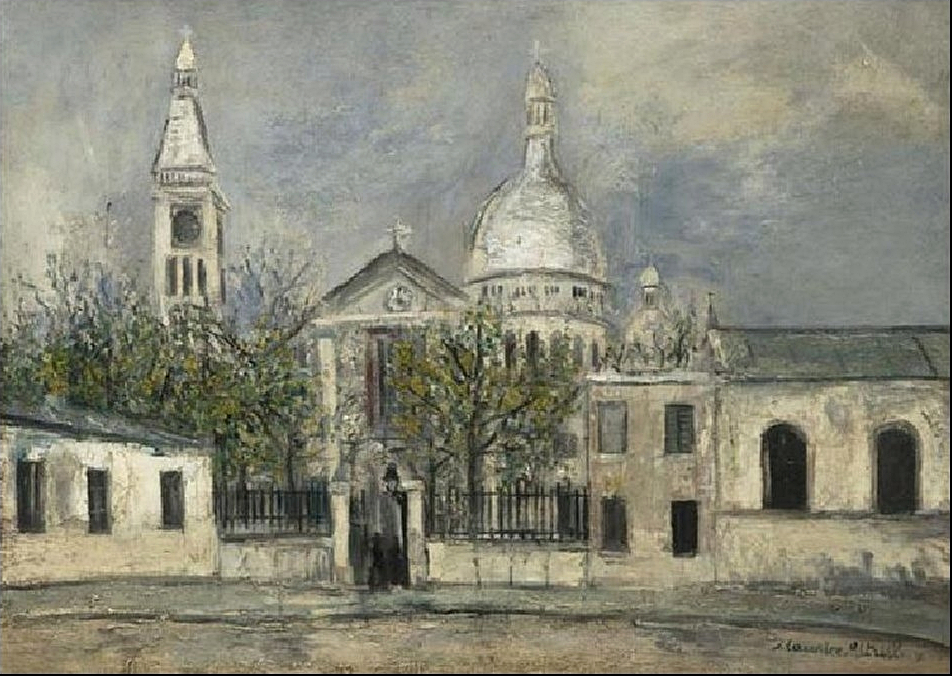This detailed painting depicts an old-fashioned, white church or government building as the central focus. The building features a distinctive grayish dome-shaped roof at the front, numerous windows with curved tops set in concrete walls, and a clock tower with a pointy steeple to the left. The scene includes a mixture of verdant greenery with dark brown tree trunks and green leaves, planted at the base of the buildings. A black wrought iron fence and gate mark the entrance, where a person in a black hat and coat or cape is seen walking forward. To the left, another smaller white building with three windows adjoins the main structure, partially concealed by more trees. The foreground shows a concrete road or walkway leading up to the entrance, flanked by two columns or posts. The sky above is a foreboding steel gray, tinged with hints of dark blue, adding to the atmospheric mood of the painting.